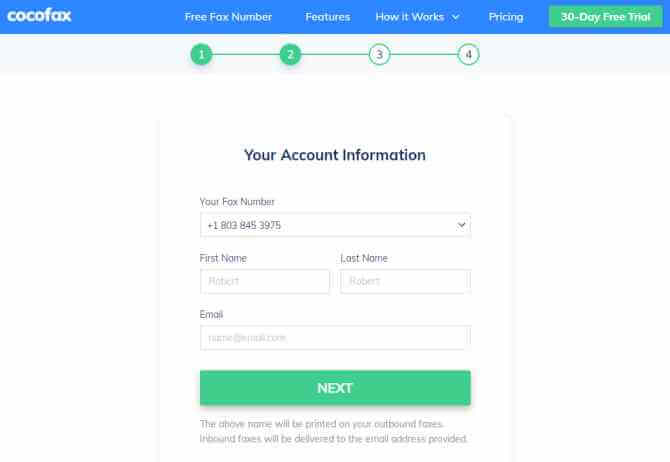This image displays the second step of a four-step registration process on the Cuckoo Fax website. At the top of the page, there's a navigation bar featuring menu options such as "Free for 30 days," "Features," "How It Works," a dropdown menu, and "Pricing." Notably, in the top right corner, there's a green bar with white text offering a "30 Day Free Trial." 

The main section of the page focuses on account information entry fields, including titles for the user's fax number, first name, last name, and email address. Below these fields, there is a "Next" button, accompanied by text indicating that the names entered will appear on outbound faxes, and that inbound faxes will be sent to the provided email address. The page header displays the service name, "Cuckoo Fax," prominently on the top left against a white background.